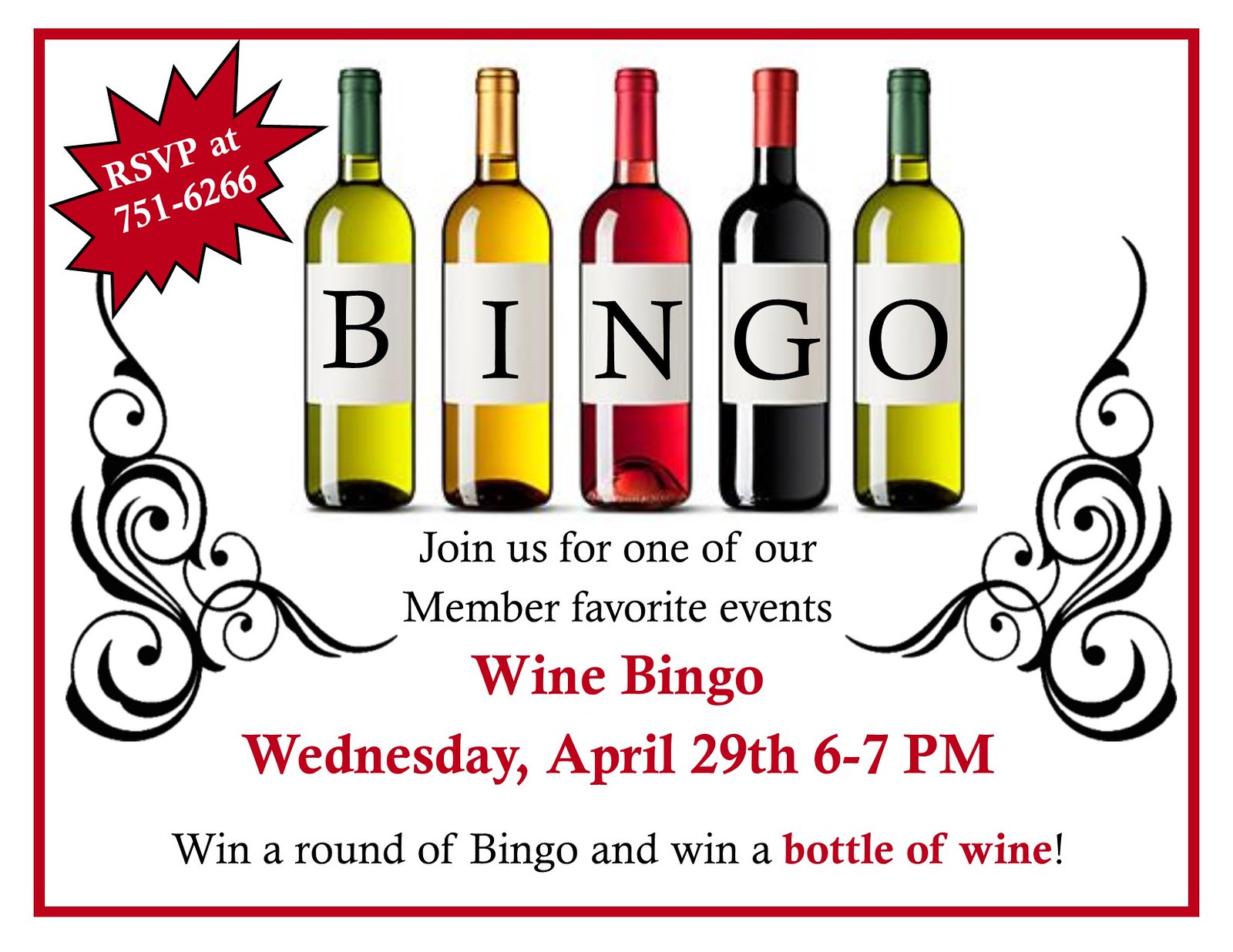This advertisement features a vibrant, rectangular design with a bold, red border and a white background. At its center, five wine bottles of various colors—green, yellow, red, black, and light green—are lined up, each displaying a letter that collectively spells out "BINGO." Above the bottles, in the upper left corner, a red starburst shape contains the white text "RSVP at 751-6266." Flanking the wine bottles on both sides are stylish black, wavy circular designs, adding a decorative touch to the layout. Beneath the bottles, the advertisement invites readers to "Join us for one of our member favorite events," and highlights in red text: "Wine BINGO, Wednesday, April 29th, 6-7 p.m." At the bottom, the text promises participants, "Win a round of BINGO and win a bottle of wine!" The overall design is a vivid blend of graphic typography and color illustration.